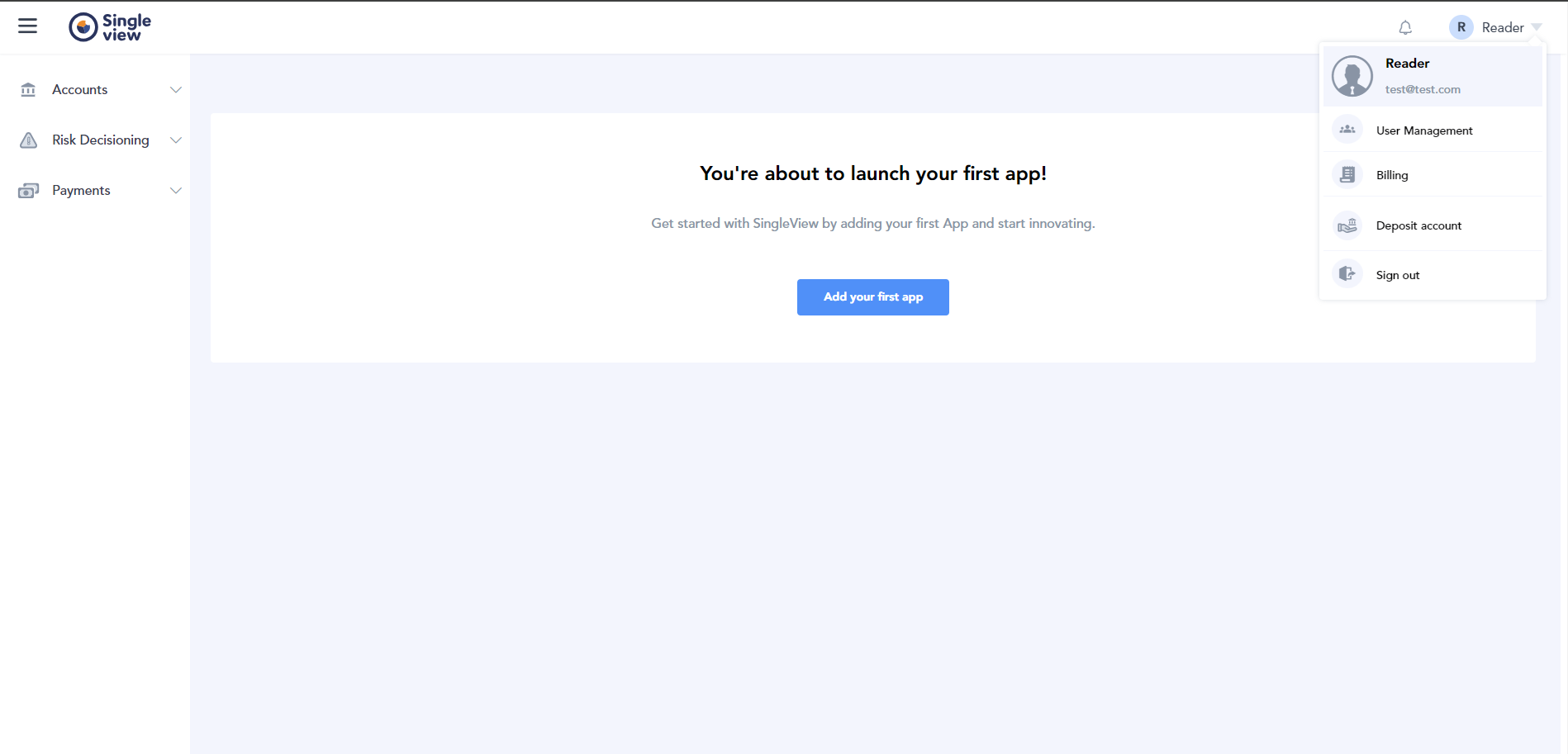The website displayed is a wide interface without a clear border, characterized by a thin black line spanning the entire top. In the upper right corner, the familiar 'hamburger' menu icon (three horizontal lines) is visible, followed by an icon indicating a single view mode, labeled "Single Top View." Just to the right is an alert icon, adjacent to a 'Reader' mode option indicated by an 'R' icon and a drop-down button. The drop-down menu reveals five options, currently highlighting 'Reader,' with additional selections for user management, other tasks unclear from the text, and a sign-out option, all in small, hard-to-read text.

Below these elements on the far right are three more options labeled 'Accounts,' another unreadable option, and 'Payments,' each accompanied by an icon to their left and drop-down arrows to their right. Dominating the central part of the screen is a light bluish-gray box, wherein a smaller white box nearly spans the width. This white box contains a centered message: "You are about to launch your first app," followed by smaller descriptive text. At the bottom of this white box, a prominent blue button invites the user to "Add Your First App."